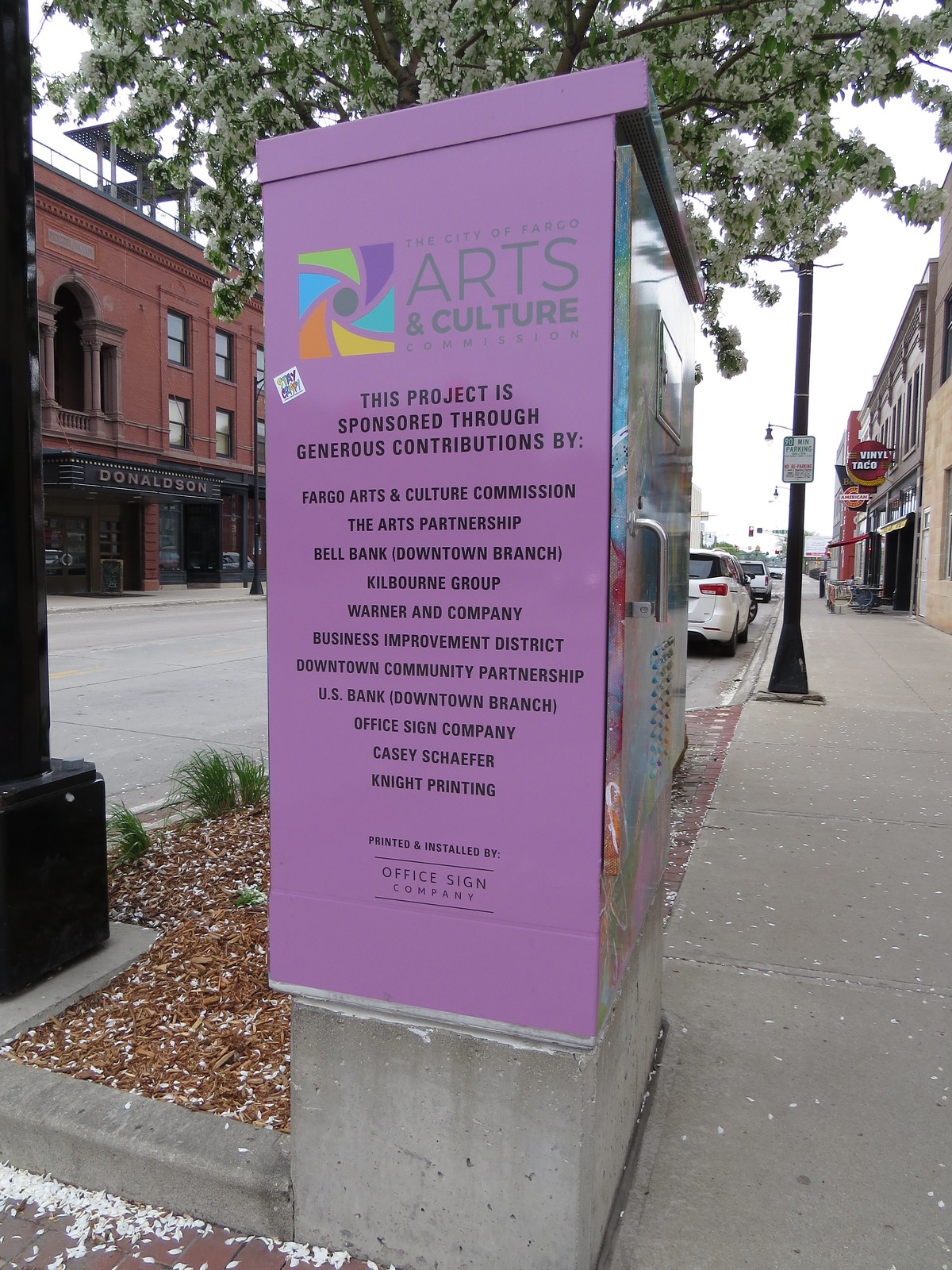The image portrays a lively city street scene, highlighted by a central purple poster proclaiming "City of Fargo Arts and Culture," positioned prominently on a metal or concrete column. This poster is adorned with a colorful square logo and acknowledges sponsorships from multiple contributors, including the Fargo Arts and Culture Commission, the Arts Partnership, Bell Bank, Downtown Branch, Kilbourne Group, Warner & Company, Business Improvement District, Downtown Community Partnership, U.S. Bank, Downtown Branch, Office Sign Company, Casey Schaefer, Knight Printing, and features an additional note stating it was printed and installed by Office Sign Company. The scene features a sidewalk on the right side of the road, with buildings lining both sides of the street and cars parked along the curb. In the background, a dark red building can be seen on the upper left, and a flowering tree peeks out from behind where the purple sign stands. The image captures a daytime setting under a clear sky, with colors such as brown, white, gray, black, green, purple, light blue, orange, and yellow punctuating the urban landscape.